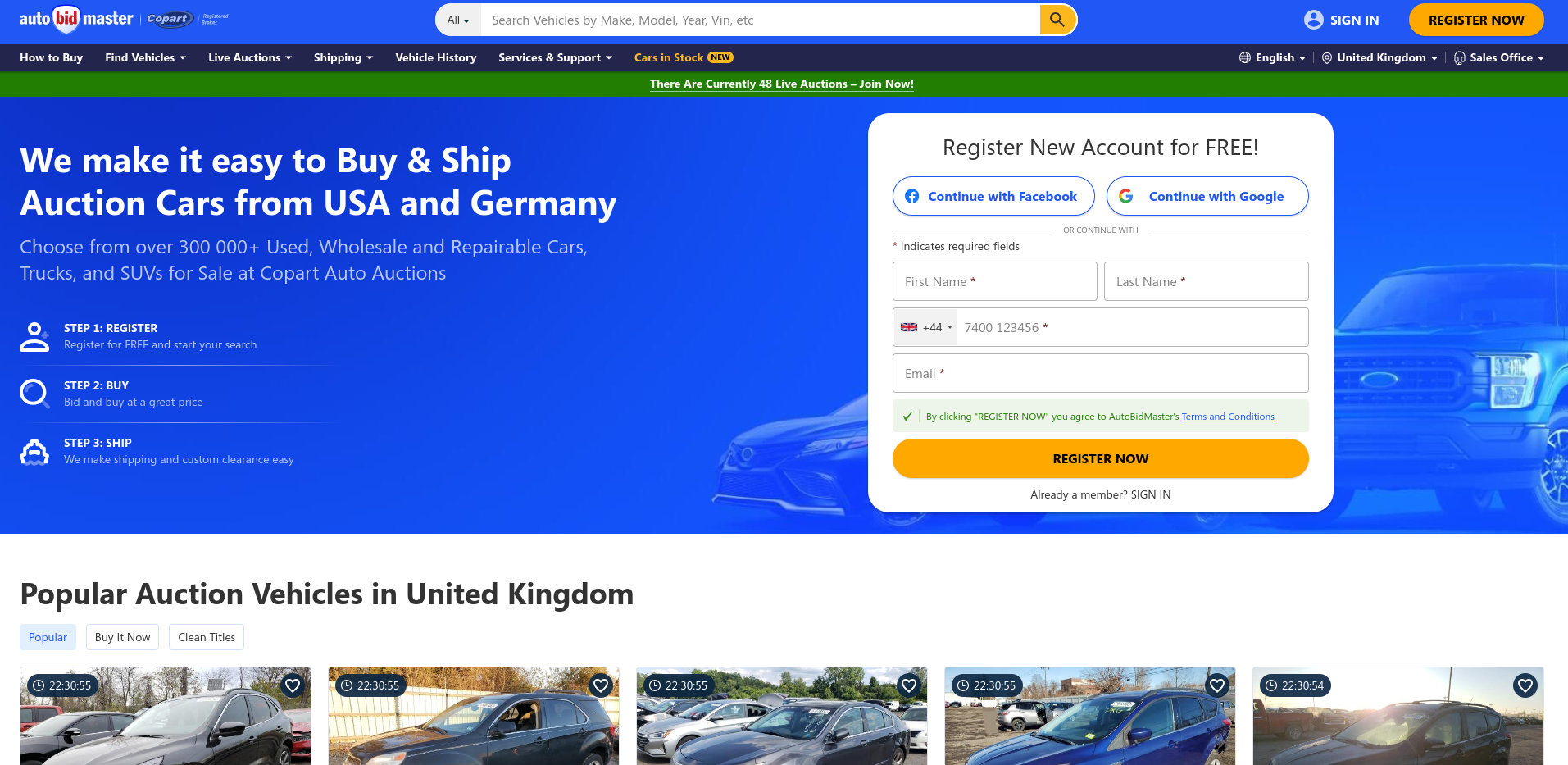The screenshot depicts the homepage of the AutoBidMaster website, a platform enabling United Kingdom residents to purchase cars from auctions in the United States and Germany and have them shipped. Dominating the top of the page is a navigation bar featuring the AutoBidMaster logo on the far left, adjacent to the Copart logo. Most of the bar's central section is dedicated to a comprehensive search function that allows users to find vehicles by make, model, year, number, and more. On the far right of this bar, there are options to sign in or register.

Beneath the main navigation bar, another banner displays various tabs for navigating the website. These tabs include 'How to Buy', 'Find Vehicles' with a dropdown, 'Buy Auctions' with a dropdown, 'Shipping' with a dropdown, 'Vehicle History', 'Services and Support' with a dropdown, and a newly added 'Cars and Stock'. To the right of these tabs, there are settings for selecting the website language (currently English), location (set to the United Kingdom), and a 'Sales Office' option.

Below this banner, a temporary notice indicates there are currently 48 live auctions in progress, inviting users to join. The bulk of the image focuses on the 'Register Now' section. On the left side, there is a message highlighting how AutoBidMaster facilitates the ease of buying and shipping auction cars from the United States and Germany. It outlines the steps necessary to set up an account and acquire a vehicle. On the right side, there is a registration form requiring the user's name, phone number, and email address, with additional options to register using Facebook or Google accounts.